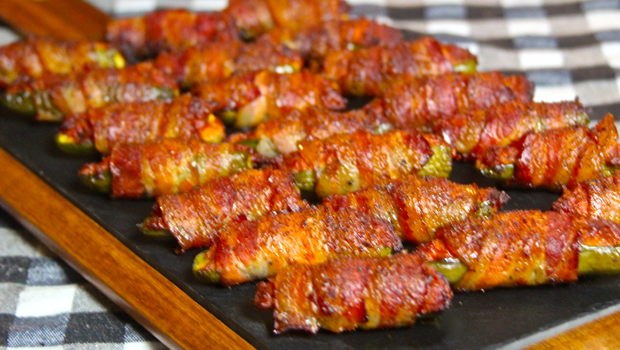This horizontal rectangle photograph prominently features a cutting board laden with bacon-wrapped jalapenos, arranged diagonally in three rows, with each row containing seven pieces. The cutting board is crafted from a brownish-tan wood with a visible grain, encased in a white border, and topped with a sleek black surface. A handle extends from the top right, pointing towards the top left. The bacon-wrapped jalapenos exhibit a medley of colors—reddish hues mixed with yellow and brown, indicative of being cooked. The background reveals a black, gray, and white plaid tablecloth peeking out at the bottom left and top right corners. The overall lighting comes from the right side, casting a natural glow on the savory appetizers, emphasizing the southwestern style of the dish. The image is contemporary, likely taken within the past 20-25 years.